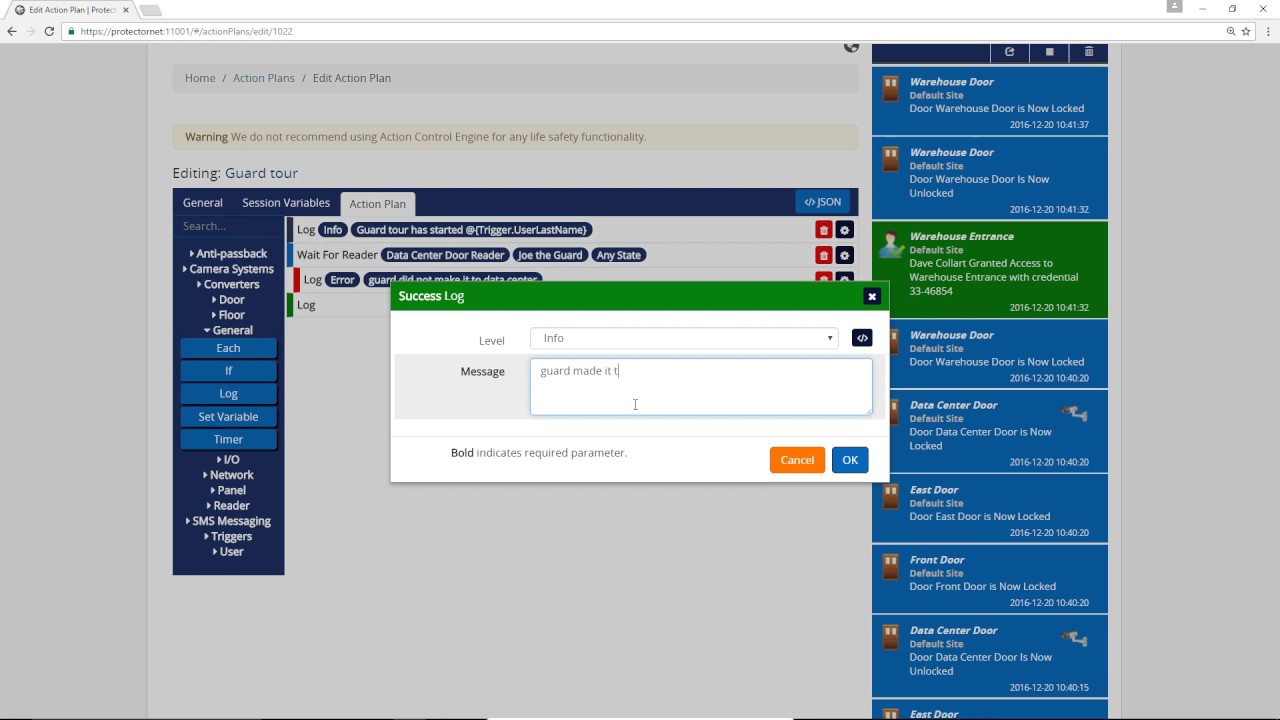This image displays an interface designed to edit an action plan, specifically named "Guard Tour," within a security or monitoring system. The screen is organized into distinct sections, each dedicated to a specific function within the action plan setup. 

1. **General, Session Variables, and Action Plan Tabs**: 
   - The **General** tab provides essential information regarding the settings related to the action plan.
   - The **Session Variables** tab contains parameters and variables that will be utilized throughout the action plan.
   - The **Action Plan** tab serves as the main working area where conditions and operations are defined.

2. **Warning Message**:
   - A prominent warning message is displayed at the top of the interface, cautioning against the use of the action control engine for life safety functionalities. This advisory indicates that the system is not intended for critical emergency response situations.

3. **Action Plan Editor with Log Entries**:
   - The action plan editor section features log entries to document actions and events. The first log entry records the commencement of the Guard Tour, categorized with an informational log level.